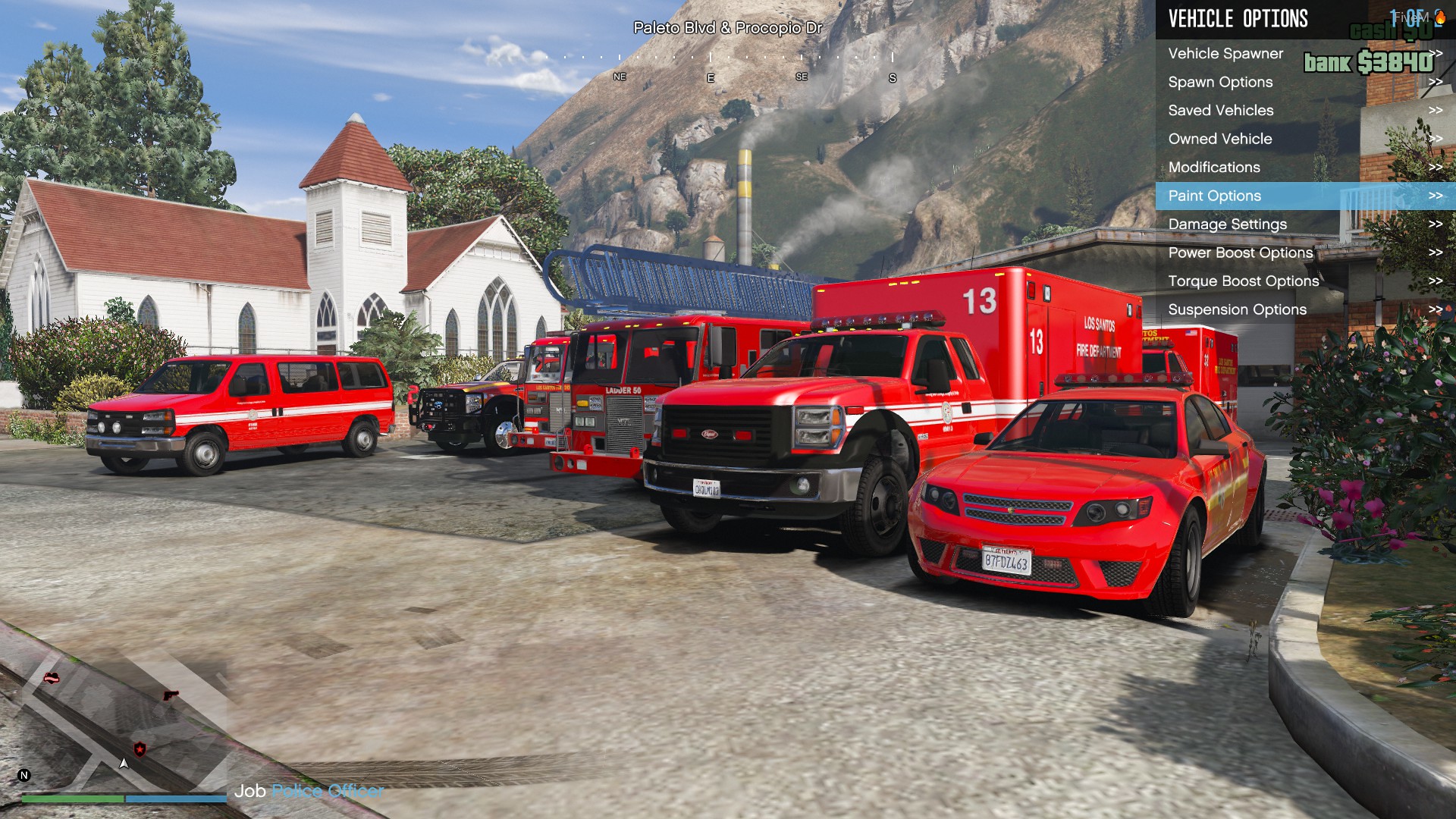The image is a color, computer-generated graphic depicting a lineup of various red emergency vehicles parked beside a white church with a red roof and arched, stained-glass windows, located under a clear blue sky. The arrangement includes a red sporty car with lights similar to a police car, two red fire trucks (the second with a prominently visible ladder), a red ambulance marked with the number 13, a red pickup truck with a canopy featuring side windows, a red van, and an additional rescue vehicle resembling an ambulance at the back. All these vehicles share a consistent red color, with some having white stripes or markings. Behind the church, you can see smokestacks emitting smoke and a towering, rocky mountain interspersed with trees. In the top right corner of the image, options related to vehicle customization and performance settings are displayed, suggesting that this graphic might be part of a simulation or a game interface.